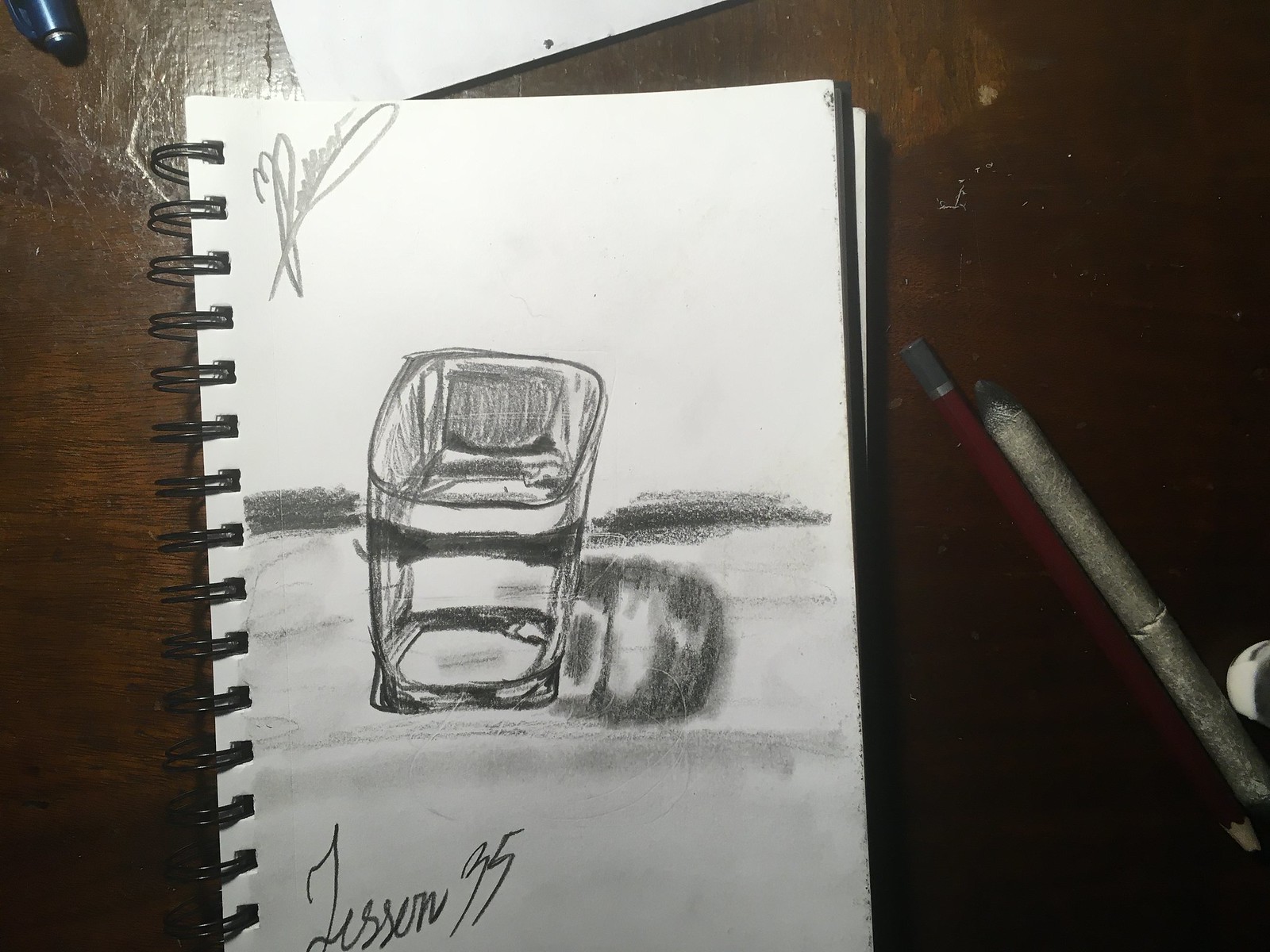This is a detailed sketch presented on white binder paper, featuring the artist's signature in the top left corner, though it's not clearly legible. On the bottom left, the text "Lesson 35" is inscribed. The drawing itself is of a container, possibly a shot glass or a trash can, depicted as standing upright, perhaps adjacent to a rock, all placed on a plain white surface. The artist has utilized pencil shading techniques, such as rubbing the pencil sideways to achieve broad and lighter lines, and has also included the container's shadow in the illustration. The paper is part of a notebook with black spirals on the left side. Additionally, to the right of the notebook, there is a red pencil with a gray tip and a piece of gray chalk. The entire scene is set on a round table, with the lighting source, likely positioned towards the top left, illuminating the sketch.